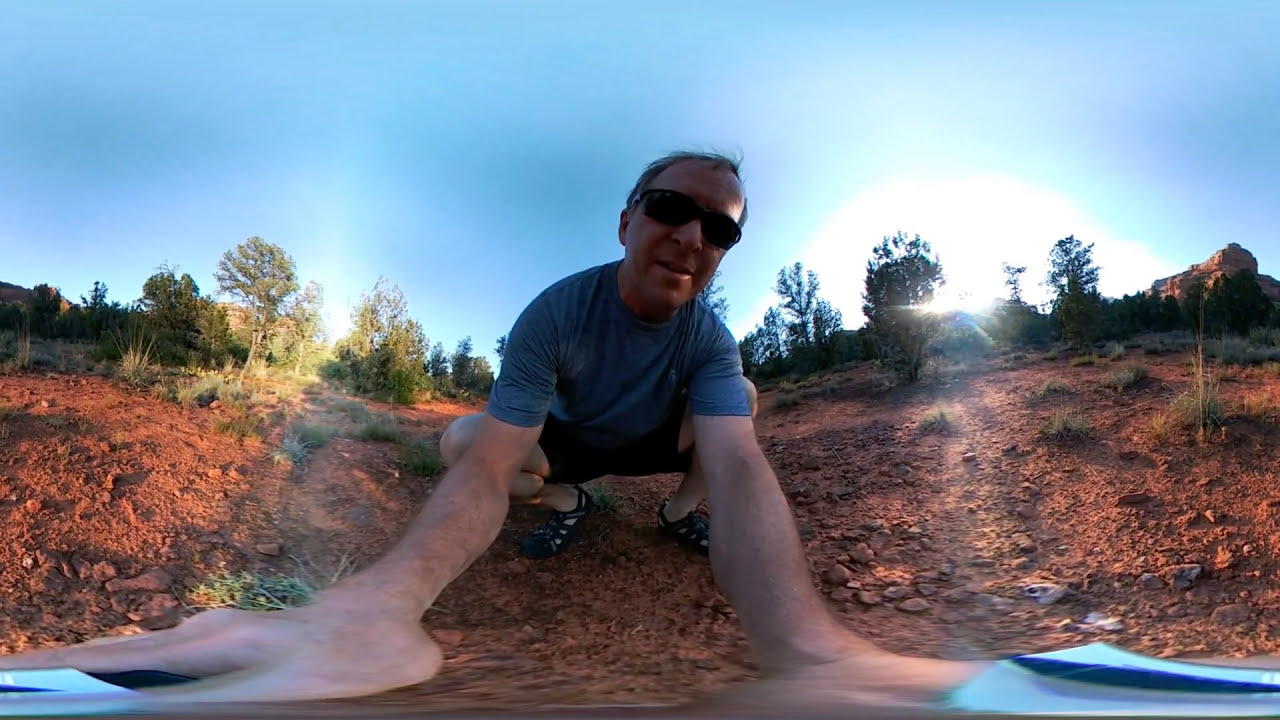An elderly man, appearing to be in his 60s or 70s, is captured taking a selfie on a red, rocky terrain that resembles a dirt or clay surface with numerous gray stones scattered about. He is squatting down, with his arms outstretched towards the camera, resulting in a wide-angle perspective that mildly distorts the image, giving his arms a slightly curved appearance. The man has short, receding dark brown to blondish hair and is wearing dark sunglasses. He sports a bluish-gray short-sleeved shirt, black shorts, and black Keen-style sandals. 

The image is set outdoors under a clear, gradient blue, cloudless sky with a large sun flare and a faint blue aura appearing in the top right quadrant. Surrounding him, there is various desert vegetation, including patches of grass, green bushes, and trees, visible on the horizon. There are no buildings or vehicles in sight, highlighting the natural, untouched landscape. The scene seems to be captured in the middle of the day, given the bright lighting and the sun's position.